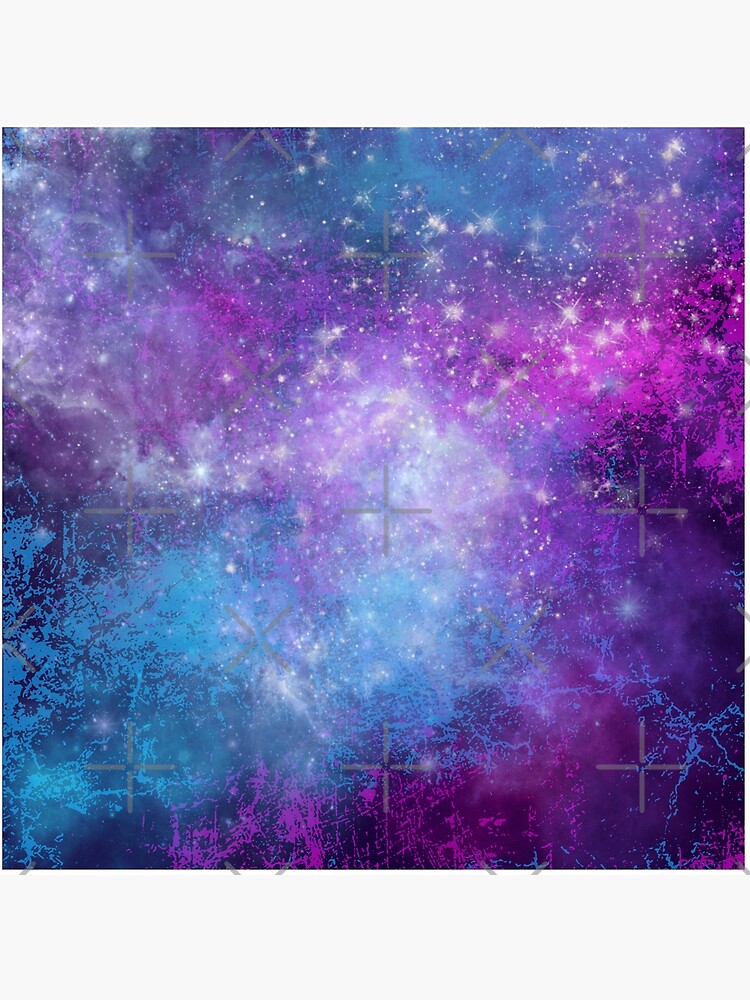This image, likely AI-generated, resembles a vibrant and abstract representation of a night sky or galaxy. The backdrop is a fusion of purples, blues, pinks, and whites, creating an ethereal, cloud-like pattern. The stars are depicted as white smudges or silver points irregularly spaced across the canvas, enhancing the dreamlike quality of the scene. Noteworthy and peculiar are the nine gray plus signs, symmetrically arranged in a 3x3 grid overlaying the image. These plus signs vary in readability and might serve as watermarks or positioning guides, adding a layer of intrigue. The overall effect is a visually striking composition that blurs the line between traditional art and digital creation.